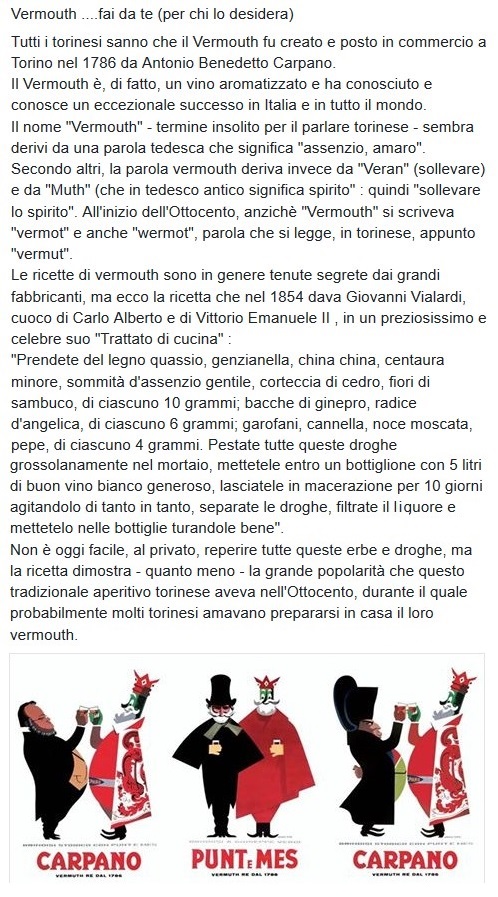The image features a long passage of text in Italian, predominantly using dark blue or black print on a white background. This text begins with the word "Vermouth" and proceeds with "fai da te," seemingly delving into the history of Vermouth from its inception around 1786 in Torino. The page comprises several paragraphs narrating this historical account. Toward the bottom of the page, there are three distinct illustrations that look like clipart images depicting characters in whimsical attire. 

In the first illustration on the left, a man with a large gut, wearing a black tuxedo jacket and possibly glasses, is toasting with a figure reminiscent of a card game's king, clad in red and white robes and a cape—this image is labeled "Carpano." The middle illustration features two more characters: one resembling a joker or king with a green face and a pointy crown, and another man in a black top hat and cape; this is labeled "Punt e Mes." The third illustration, like the first, is labeled "Carpano," again showcasing two characters enjoying a drink together. Each illustration underscores the theme of drinking and celebrating with Vermouth.